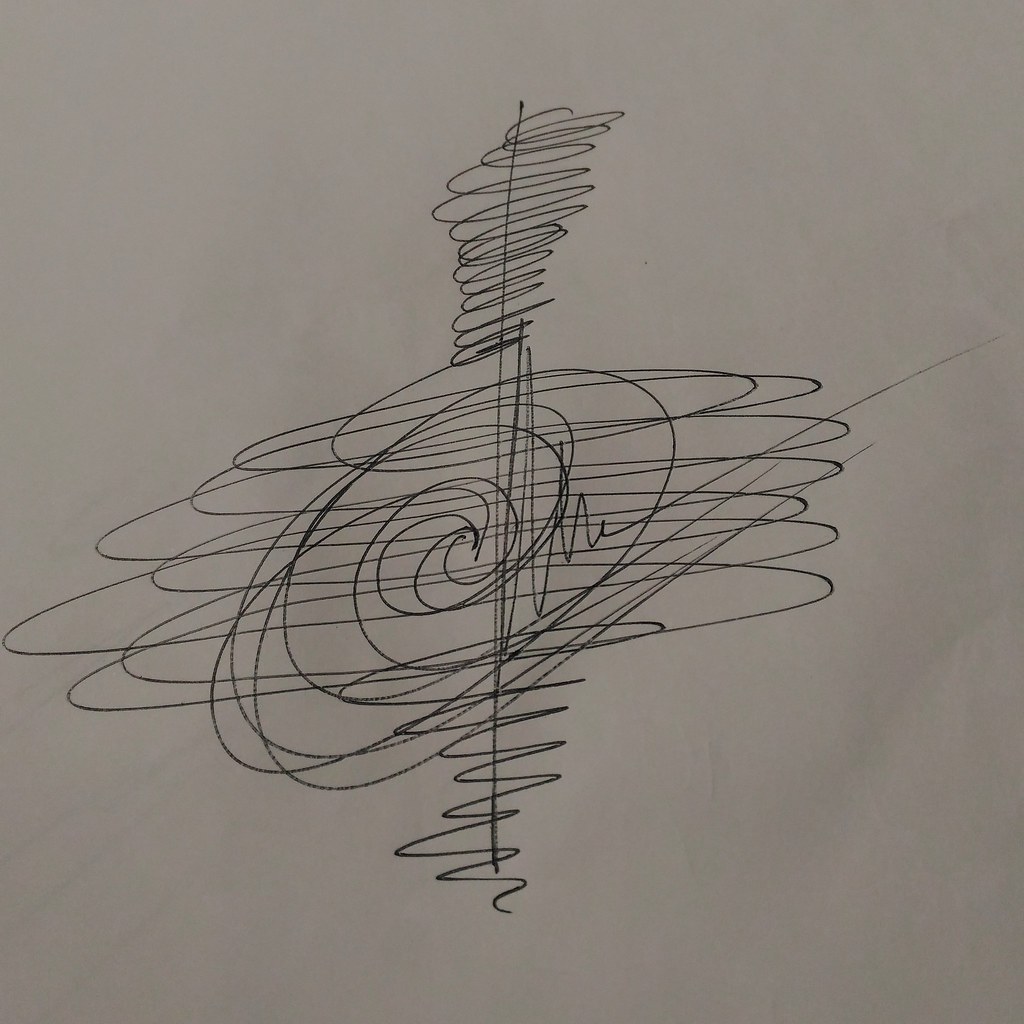This image captures a photograph of a white piece of paper, likely taken in an indoor setting. The white paper serves as the canvas for an intricate black pen drawing. The drawing features an array of geometric elements, including multiple lines and circles, with a prominent straight line running vertically down the middle. Additionally, there are several spiral patterns that extend both horizontally and vertically across the paper. The overall composition appears simple and straightforward, with the stark contrast between the black ink and the white background emphasizing the design. The photograph itself is rectangular in shape, framing the artistic interplay of lines and shapes neatly within its bounds.